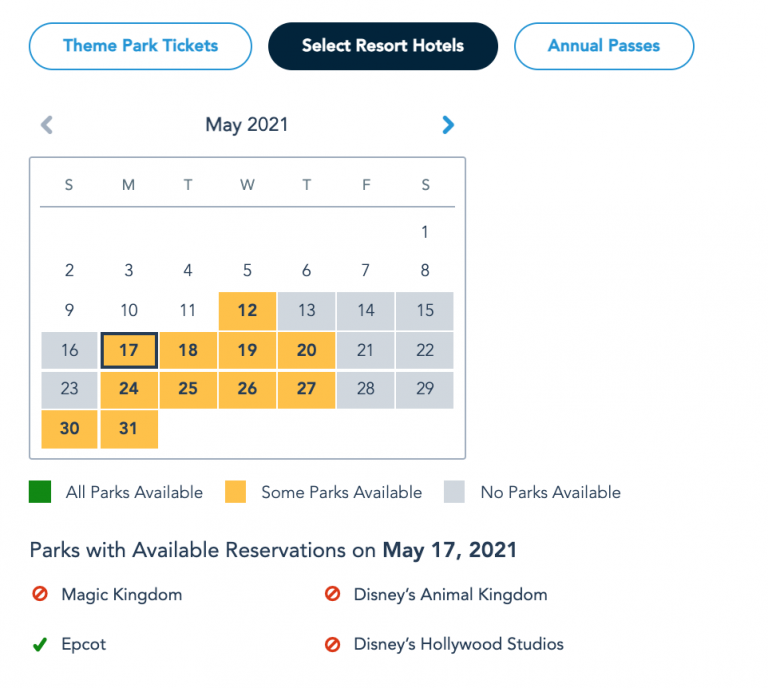The image depicts a date selection interface for booking theme park tickets, selecting resort hotels, and viewing annual passes. At the top, there are three buttons: "Theme Park Tickets," "Select Resort Hotels" (which is currently selected), and "Annual Passes." The calendar is displayed for May 2021, with navigational arrows on either side to switch months. The days of the week run horizontally across the top, and individual dates follow below. 

Specifically, Monday, the 17th of May, is highlighted as selected. Several dates, including May 12th, 17th, 18th, 19th, 20th, 24th, 25th, 26th, 27th, 30th, and 31st, are marked in yellow, indicating partial availability. Dates following the 12th that are not yellow are shown in grey, meaning no availability.

A legend at the bottom explains the color coding: green signifies all parks available, yellow indicates some parks available, and grey denotes no parks available. Below this key, there's a note indicating "Parks with available reservations on May 17th, 2021." Next to it, symbols indicate the availability: Magic Kingdom, Disney's Animal Kingdom, and Disney's Hollywood Studios each have a circle with a slash, showing no reservations available. Epcot, marked with a checkmark, is the only park with available reservations.